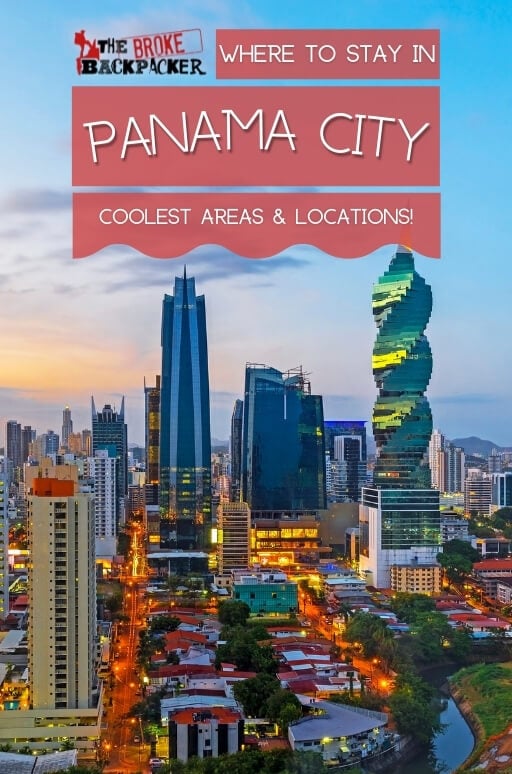The image appears to be a vibrant travel poster promoting Panama City. The text on the poster enthusiastically invites travelers with the headline, "Where to Stay in Panama City? Coolest Areas and Locations!" Below this, the tagline "The Broke Backpacker" suggests that the guide is tailored for budget-conscious solo travelers or groups seeking affordable yet exciting experiences in Panama City.

The poster features a stunning skyline, capturing a mix of modern skyscrapers and charming low-rise buildings, all illuminated by the warm hues of a sunset. One notable architectural highlight is a uniquely designed building that spirals upwards, showcasing the city's innovative style. The overall scene presents a dynamic urban landscape filled with lights and bustling life, enticing viewers to explore the diverse and lively neighborhoods of Panama City.